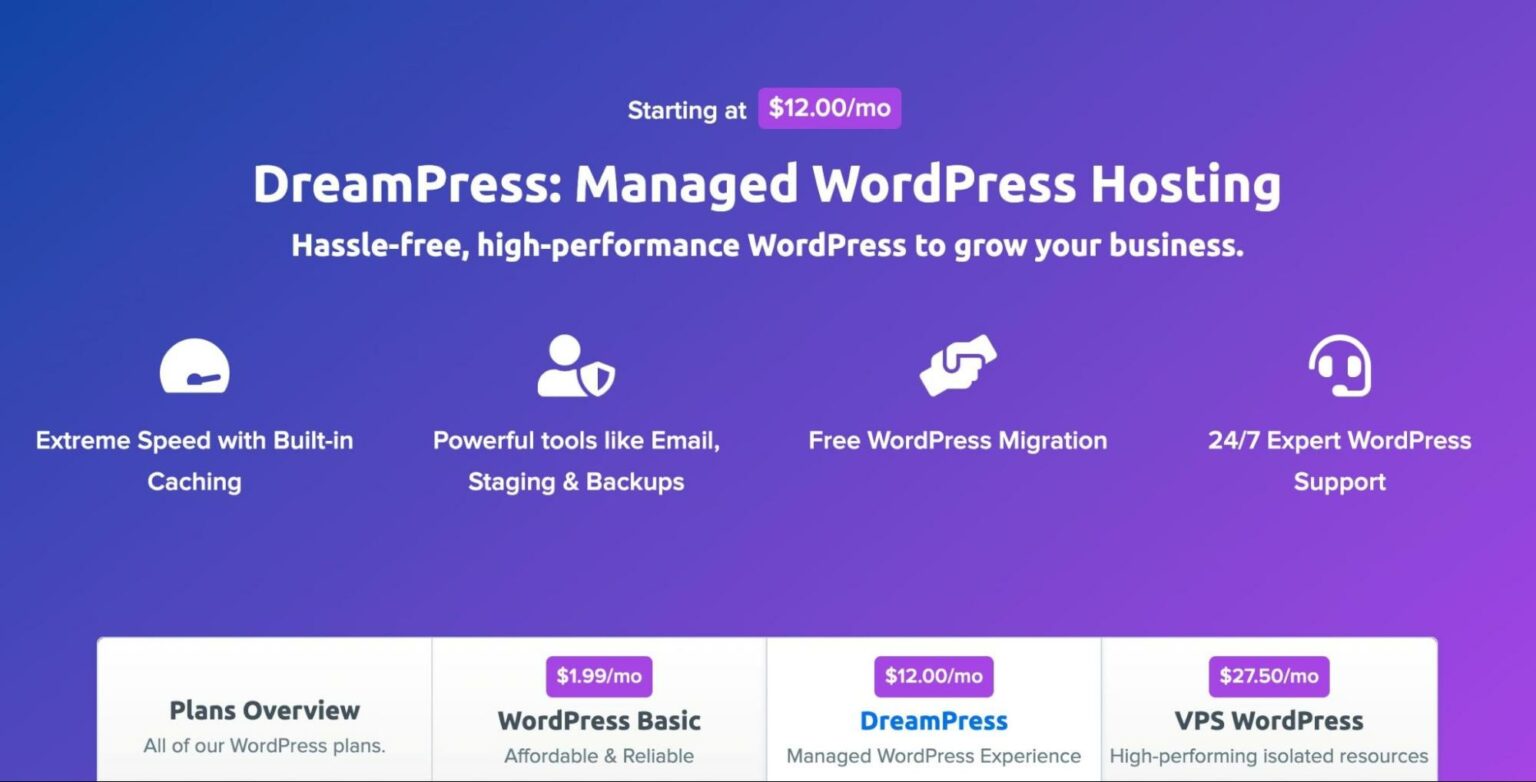The home page for DreamPress presents an inviting and well-structured overview of their managed WordPress hosting services, starting at $12 per month. The top section prominently displays this price on a vibrant pink background. The headline reads "DreamPress Managed WordPress Hosting," emphasizing its hassle-free, high-performance solutions designed to help grow your business.

Beneath the headline, there are four informative icons with corresponding features:
1. A full speedometer symbolizing "Extreme Speed" with built-in caching for faster performance.
2. A human figure with a shield representing "Powerful Tools" such as email staging and backups.
3. Two hands shaking, indicating "Free WordPress Migration" services.
4. A pair of eyes with a headset, denoting "24/7 Expert WordPress Support."

At the bottom of this section lies a large white rectangle featuring four additional options: 
- Plans Overview
- All Your WordPress Plans

Below these, there are buttons for three different plan options:
1. "WordPress Basic" priced at $1.99 per month, with white text on a purple button, highlighting affordability and reliability.
2. "DreamPress" at $12 per month, labeled in blue, advertising a managed WordPress experience.
3. "VPS WordPress" costing $27.50 per month, promoting high-performance and isolated resources.

The entire layout is set against a gradient background that transitions smoothly from blue in the upper left corner to a light lavender in the bottom right, creating an aesthetically pleasing and calming digital atmosphere.